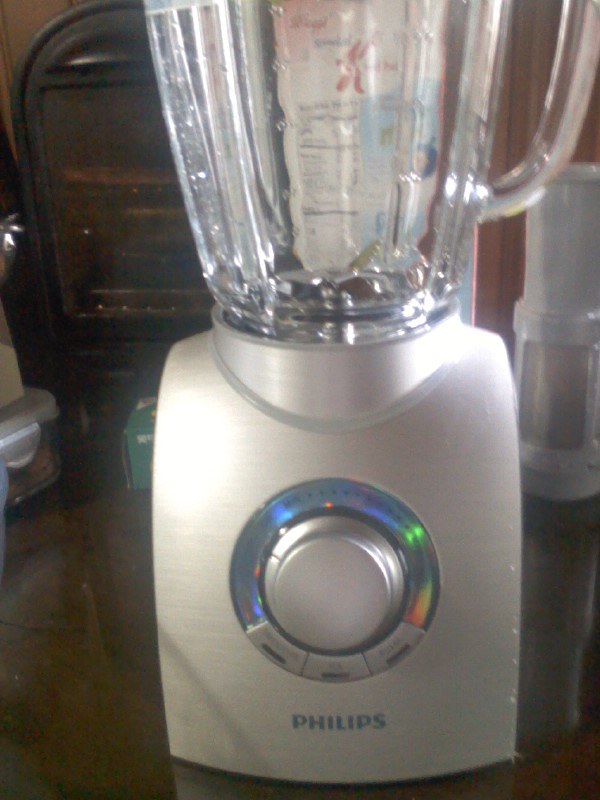This close-up color photograph, taken indoors in portrait mode, showcases a Philips blender positioned on a dark brown counter. The base of the blender is a very light silver or grayish-white color. Prominently displayed on the front of the blender is a silver rotary dial with iridescent hues of green, blue, red, and orange, encircled by gradations for selection. Below the dial, there are three buttons. The brand name, Philips, spelled P-H-I-L-I-P-S, is clearly visible below the dial. The top section of the blender features a glass pitcher with a pouring spout and a handle oriented to the right. In the background, off to the right, there are attachments and possibly another appliance, which might be a food processor or the back of a coffee maker. Additionally, the control panel of an oven and a "Special K" cereal box can be seen behind the blender. The overall lighting of the photograph is slightly dim, and the image is somewhat out of focus.